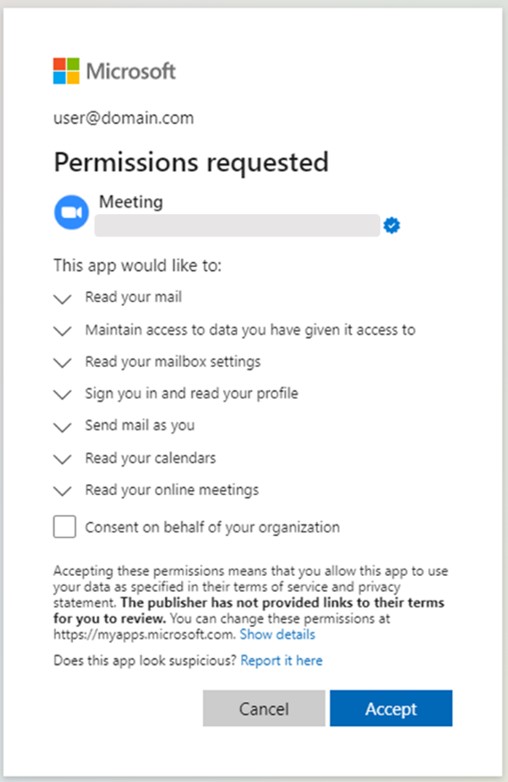The image is a screenshot taken from a computer or tablet, featuring a predominantly white background. At the very top, the familiar Microsoft logo is displayed, consisting of four small squares arranged to form a larger square. The top-left square is red, the top-right is green, the bottom-left is blue, and the bottom-right is yellow, with each square slightly separated. Next to the logo, the word "Microsoft" appears in a thick, gray font.

Below the logo, in a thinner gray font, the text "user@domain.com" is visible. Underneath this text, a large black font reads "Permissions requested." Directly beneath, the word "Meeting" is displayed next to a blue circle featuring the side profile of a white camcorder icon.

Beneath the word "Meeting," there is a very thin, elongated gray box with a cogwheel icon and a white checkmark, similar to the checkmark used on Twitter, at the end of the box. Further down, in a thinner gray font, the text "This app would like to:" is followed by a list of permissions, each with a downward-pointing arrow devoid of a tail. The list includes:
- Read your mail
- Maintain access to data you've given it access to
- Read your mailbox settings
- Sign you in and read your profile
- Send mail as you
- Read your calendars
- Read your online meetings

Below the list, there is a small checkbox labeled "Consent on behalf of your organization." A section below this outlines policies and terms of agreement. At the very bottom of the image, there are two side-by-side buttons: a gray "Cancel" button on the left and a blue "Accept" button with white text on the right.